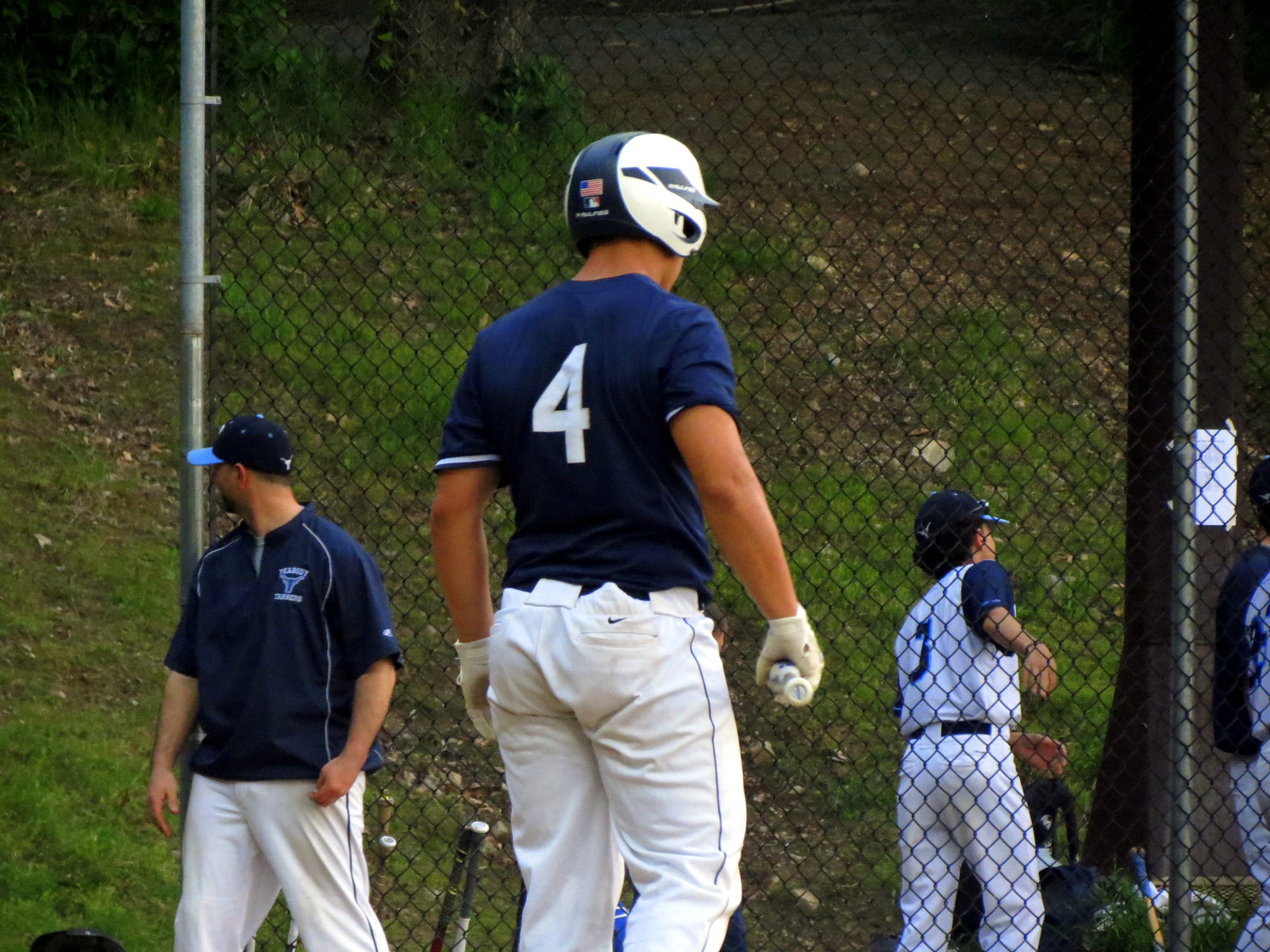In this detailed image of a daytime outdoor baseball scene, we observe three baseball players. The primary focus is on a male player in the immediate foreground, facing away from the camera. He is dressed in a navy blue uniform top with the number four in white on the back, and white pants showcasing a small blue Nike check. He wears white baseball gloves and a white and navy blue helmet adorned with an American flag emblem and possibly the National Baseball League logo.

To his left stands another male player, who is turning his head to the left. This player dons a blue baseball cap with aqua blue shading, a short-sleeved blue shirt with an indistinct logo, and white pants. Beyond them, slightly to the right, is a third player, possibly female, clad in a white jersey and white pants. This player also wears a blue baseball cap and holds a catcher's mitt.

The setting includes a tall chain-link fence typical around baseball fields to protect batters. Behind this fence, there is a grassy hillside with a dirt patch and some brush or bushes, along with a tree to the right, which has a white piece of paper taped to it. Several baseball bats are lined up against the fence, adding to the bustling atmosphere of the game in progress.